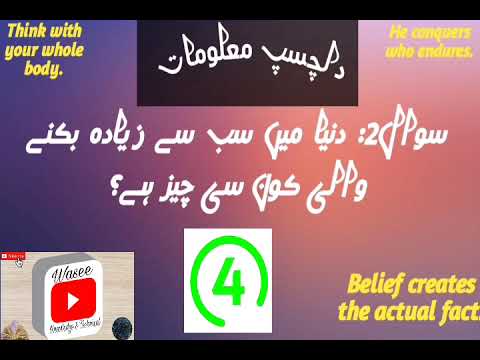This image is a colorful, motivational slide or poster with a blend of text, logos, and various colors, primarily purple that transitions into a peach-pink gradient. The design features multiple inspirational quotes. In the top left corner, yellow text on a purple background reads, "Think with your whole body." The top right shows another quote in yellow, stating, "He conquers who endures." At the bottom right, in yellow text against a lighter purple background, it says, "Belief creates the actual fact."

The slide includes several logos: a YouTube logo in a white tile situated at the bottom left corner, which also has the letters "W-A-S-E-E" above it and some unreadable text below. In the bottom center, there's a white square containing a green semicircle that partly encloses the number '4.' Scattered throughout the image, there are additional texts in a script that appears to be Middle Eastern or another unfamiliar language, prominently placed at the top center inside a black rectangle with white print, and also spread out across the background in various locations.

The background and the diverse text colors—black, yellow, blue, pink, green, red, brown, and tan—add a vibrant and dynamic feel to the slide, indicating it was likely created in PowerPoint and aimed at delivering motivational messages.